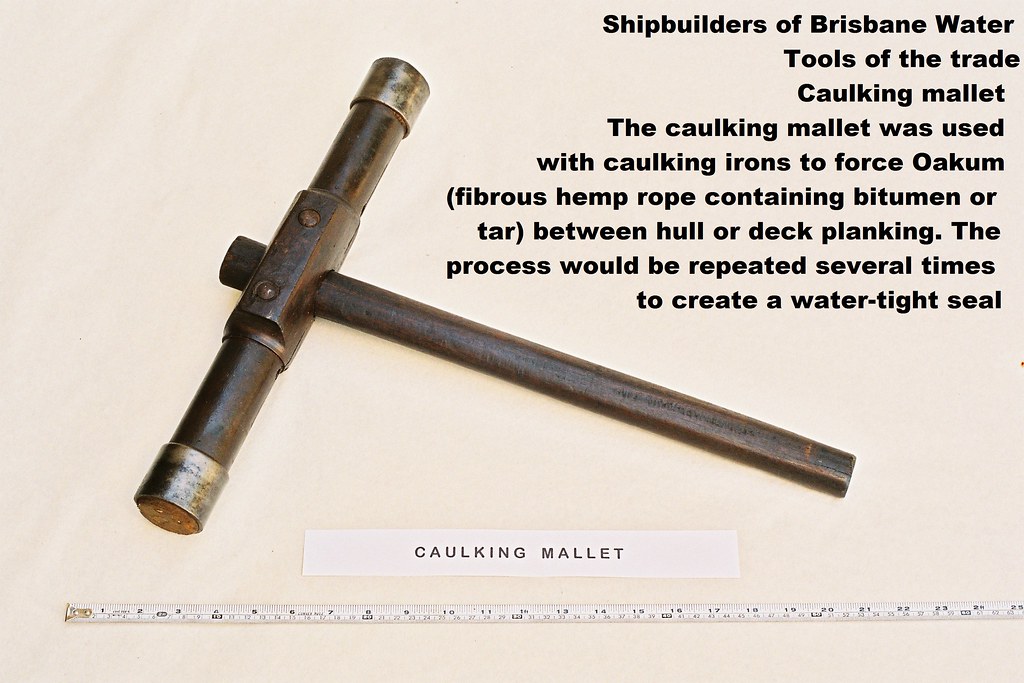The image features a caulking mallet prominently displayed against a white background. The mallet, which appears tarnished and aged, is composed of black and silver metal. It has a distinctive shape resembling a small hammer with a disproportionately long head and blunted ends, almost as long as the handle itself. Below the mallet, a black and white measuring tape stretches across the image, marked up to 25 inches, though the exact units are unclear. 

A white label below the mallet states "Caulking Mallet." In the upper right corner of the image, black text reads: "Shipbuilders of Brisbane Water — Tools of the Trade: Caulking Mallet. The caulking mallet was used with caulking irons to force oakum, fibrous hemp rope containing bitumen or tar, between hull or deck planking. The process would be repeated several times to create a watertight seal." 

The mallet's functional and historical significance is thus emphasized by its detailed description and its association with traditional shipbuilding techniques.